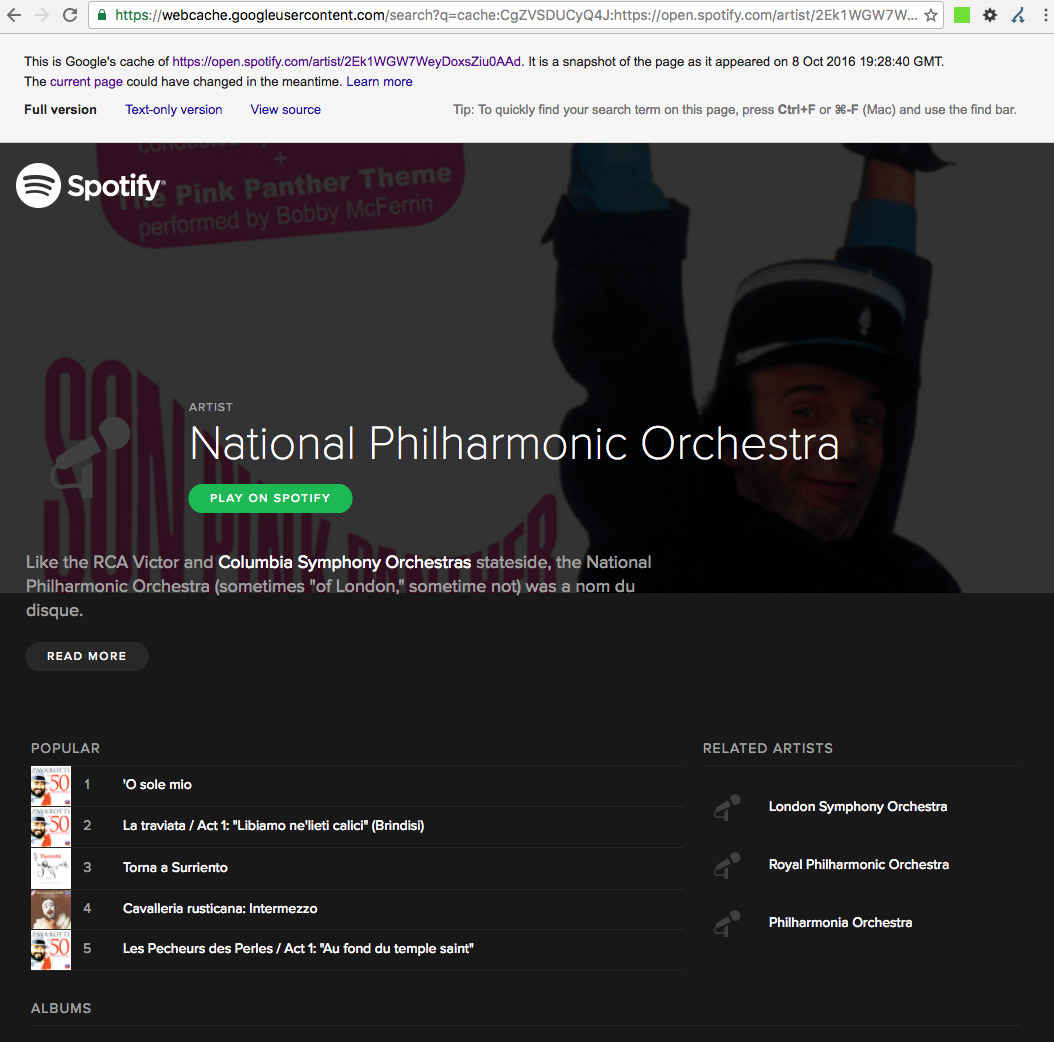This image is a screenshot of a cached webpage, specifically a snapshot of a Spotify artist page as it appeared on October 8th, 2016, at 7:28 PM GMT. The URL indicates it was retrieved from webcache.googleusercontent.com, signifying that it is a saved version of the original page. The Spotify page in question belongs to the National Philharmonic Orchestra.

The top portion of the page features a banner that partially displays an album cover, though it is not fully visible. Below the banner, there is a detailed description of the National Philharmonic Orchestra. The description highlights that, similar to the RCA Victor and Columbia Symphony Orchestra in the United States, the National Philharmonic Orchestra (sometimes noted in quotation marks as "National Philharmonic Orchestra" of London) is identified as a Nom du Disque, which is a term of French origin meaning "record name."

Further on the page, there is a listing of the orchestra's top five most popular songs according to Spotify. Additionally, a section shows related artists that listeners may be interested in. If one were to scroll down the page, they would likely encounter a catalog of the National Philharmonic Orchestra's albums.